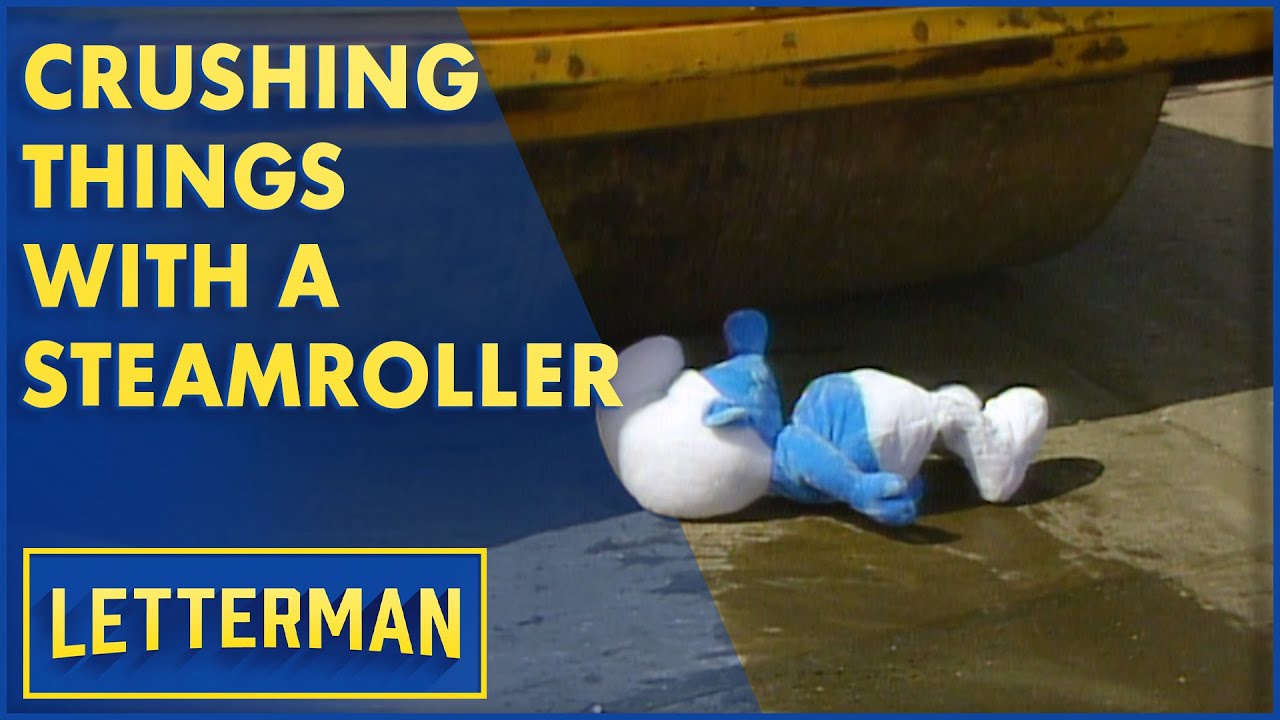In the image, a small, slightly worn Smurf plushie, about a foot tall and colored in white and blue, lies flat on a stone pavement stained with water. Hovering ominously next to the Smurf is part of a large, dark steamroller with a distinctive yellow rim, poised as if about to crush the toy. The scene is intended as a comedic segment for the Letterman show, suggested by the promotional text in bold yellow letters on a blue background in the upper left corner, which reads "crushing things with a steamroller." Additionally, the word "Letterman" appears in yellow lettering within a box at the bottom left corner of the image. The contrasting blue, yellow, and orange color scheme enhances the quirky and dramatic atmosphere of the picture.